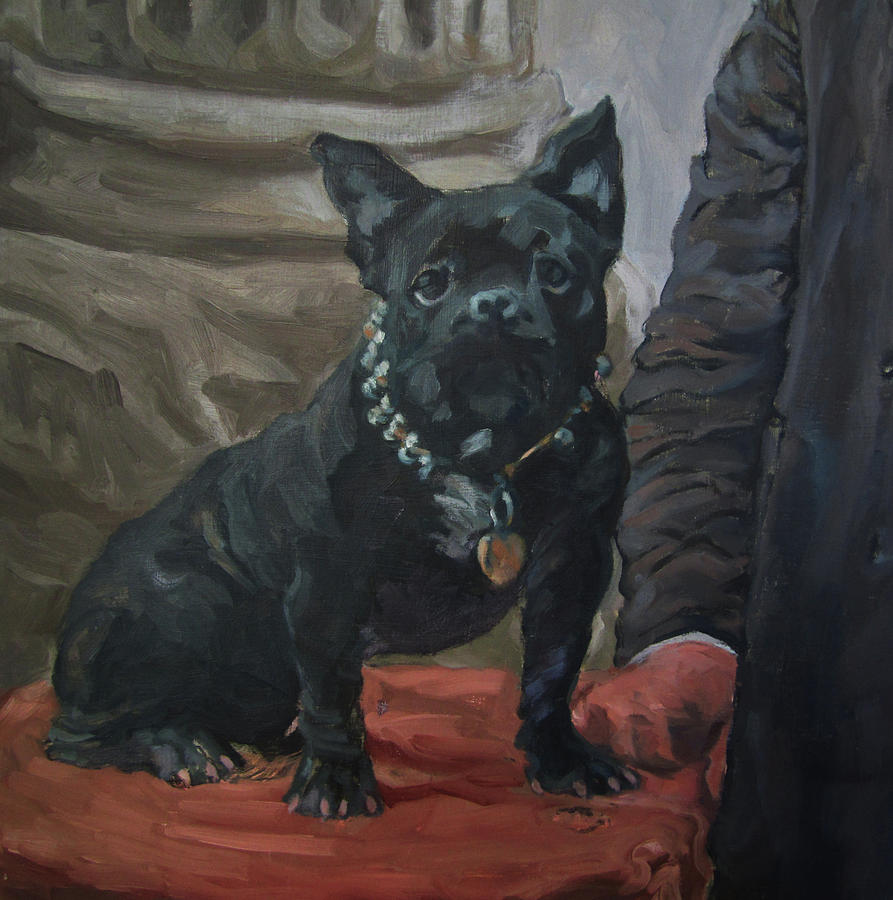The image is a square painting, rendered in an impressionistic or post-impressionistic style, characterized by loose, expressive brushstrokes and rich color. Dominating the scene is a small black French Bulldog, distinguished by its muscular build and pointy ears, likely hinting at a mixed breed. The dog sports a prominent, bulky collar with an intertwined metal and rope chain, from which dangles a heart-shaped pendant. Positioned on a red or mauvish-red cushion, the dog is perched on a pedestal or stool, raised to the level of a man's arm, which rests on the surface beside the dog. The man's arm and hand, clad in a dark coat or jacket with a glimpse of a white shirt cuff and lighter skin, are all that's visible of him, hinting at his presence without revealing his full form. The backdrop of the scene includes the base of a column, suggesting an outdoor setting, and the overall color palette features predominantly dark blues and grays, contributing to a moody and intimate atmosphere.